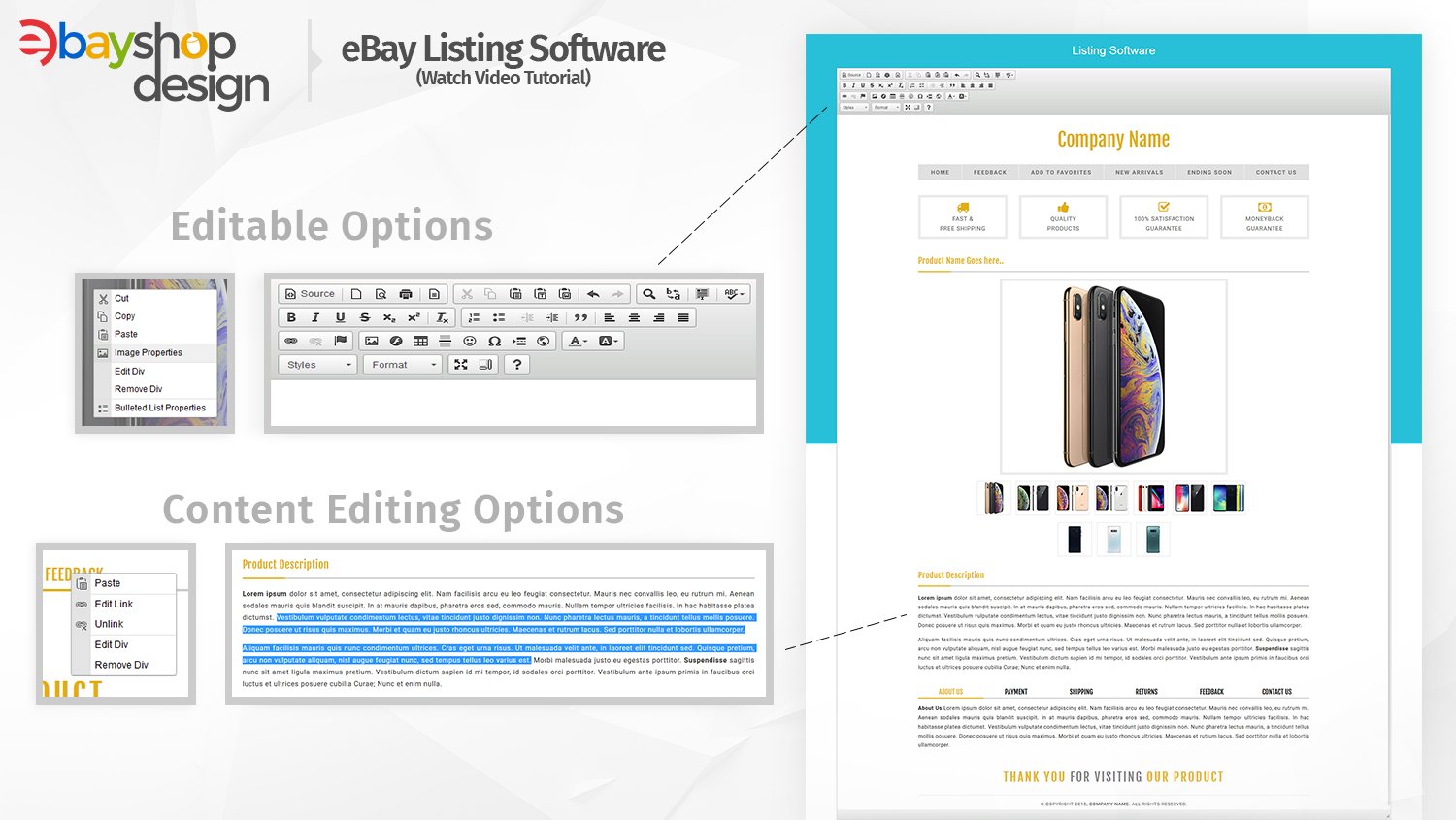This image depicts a detailed interface of a website with a predominantly gray backdrop. In the top-left corner, there's an outlined "E" with a red accent at its center. The "E" features an opening on the right with a red line extending inwards and a red border that travels upwards to the top of the outline.

Below this, the phrase "base shop" is displayed, followed by a vertical gray line. The bold black text "ebay listing software" appears prominently beneath it, with a parenthetical note that says "watch video tutorial." Further down, large gray letters spell out "edible options."

Adjacent to these elements is a square containing various commands such as "copy," "paste," and "cut out." To its right, there is a gray rectangle with a small white border at the bottom, containing multiple tabs. Below these content editing options is another small square on the left side, which holds five different options.

Nearby is a rectangle labeled "product description," describing the product in approximately eight lines of text. The right side features a dark blue border that extends halfway down the left side, across the top, and halfway down the right side. At the top of this blue border, the phrase "listing software" is displayed in white text.

Beneath the blue border is a gray section filled with icons on the left. In the center region, white text with a goldish hue spells out "company name." Below this, there are six gray tabs with black lettering, followed by four white boxes outlined in gray containing various options.

At the bottom left, the text "product name goes here" is highlighted in gold. The section also includes a prominent image of three phones arranged side by side, accompanied by approximately twelve smaller images underneath. The interface concludes with additional product descriptions, detailed information, and six more tabs at the bottom.